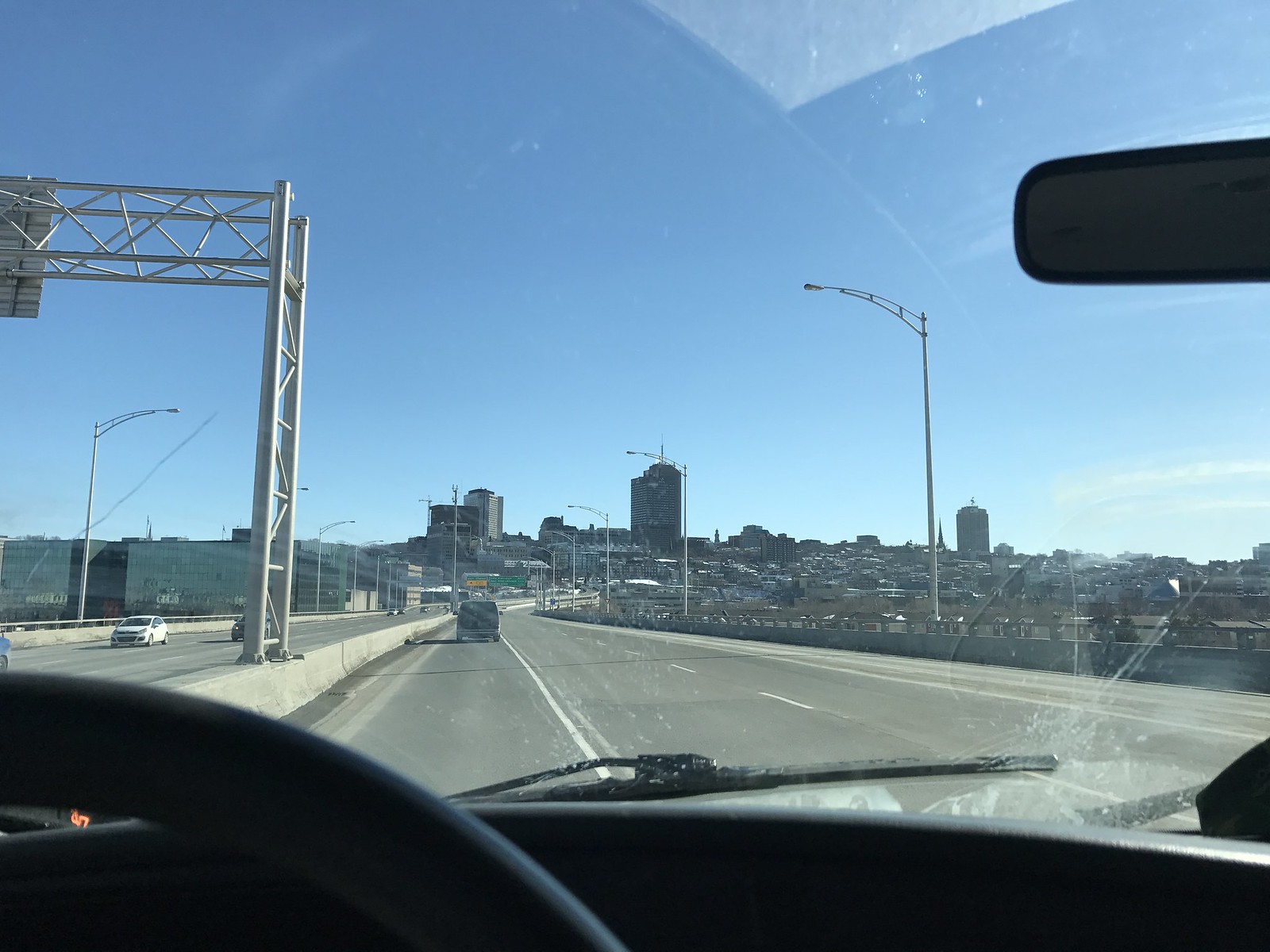This photograph, taken from the driver's seat of a moving car on an elevated highway bridge, encapsulates a vibrant urban scene on a clear, sunny midday. The driver's perspective includes a partial view of the steering wheel, spanning from 12 o'clock to 2 o'clock, along with the silhouetted dashboard and windshield wiper. The windshield is slightly dirty and reflects the bright ambient light. The car is in the left lane, demarcated by a white stripe that designates it as the high-occupancy vehicle lane, with two other lanes to the right. Up ahead, a dark-colored pickup truck is visible. The highway, divided by concrete barriers, reveals several vehicles traveling in the opposite direction and an overhead sign supported by a large gantry structure on the other side. Streetlights line the right side of the road, spaced evenly along the route. In the background, the urban skyline features three prominent tall buildings atop a hill, with numerous shorter structures dotting the landscape. The wide expanse of baby blue sky adds a serene backdrop to the bustling city scene.